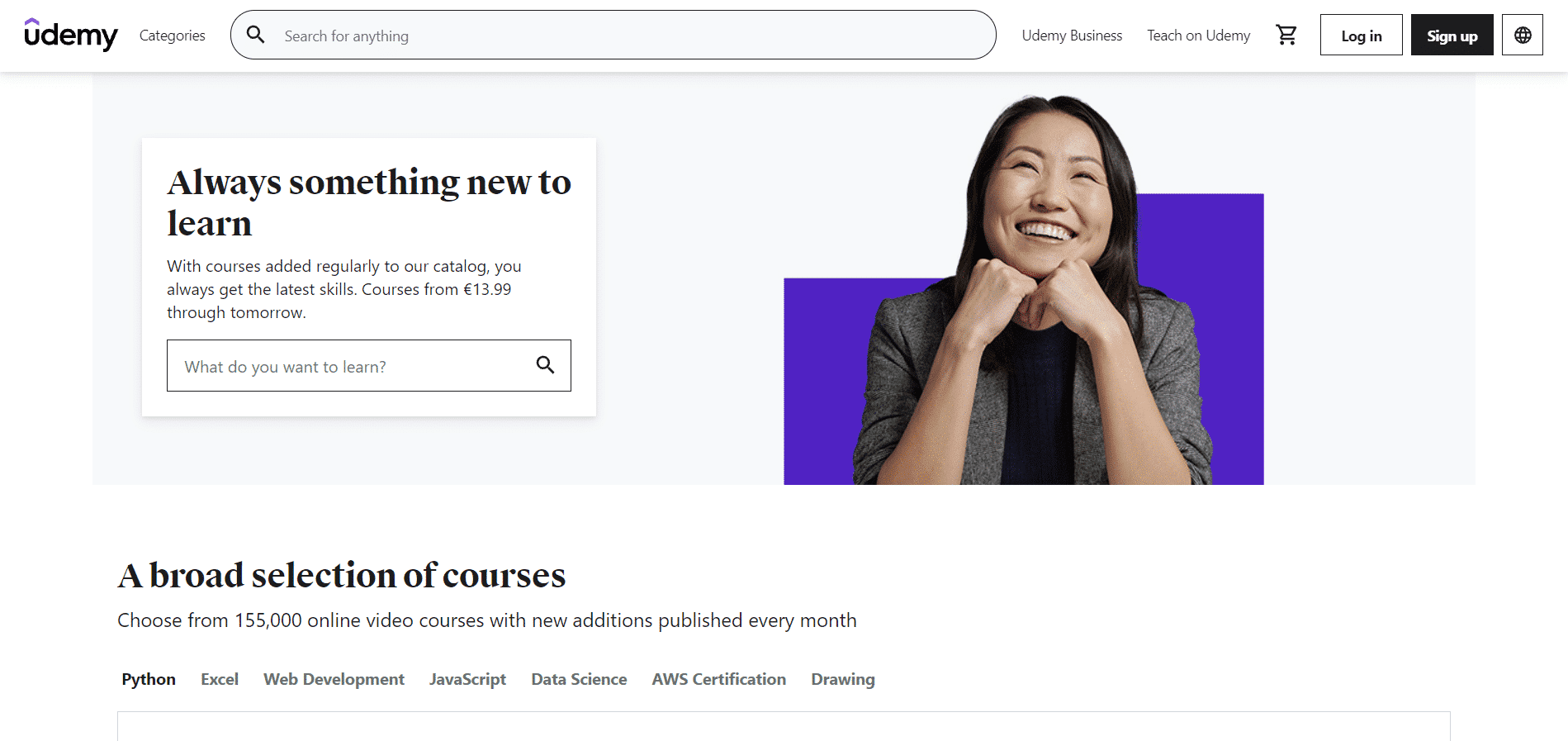This image showcases the homepage of the educational platform website, Udemy. The website's main color scheme is a clean and minimalistic white, with subtle accents to differentiate sections. At the very top of the page, a prominent search bar invites users to "Search for anything." To the left of the search bar, navigation links for various categories are listed, while to the right, there are options for "Udemy Business," and another section labeled "Tick on Udemy." The top bar also features a shopping cart icon, indicating where users can finalize their course purchases, and options to either log in or sign up for an account.

Just below the navigation bar, there is a headline with promotional messaging, encouraging users to "Always learn something new." This area also includes a support or help bar for user assistance. Beneath this, the platform highlights a broad selection of courses available, ranging from Python programming and Excel tutorials to web development. 

The only image on this page features an Asian woman with long black hair, smiling warmly at the viewer. She is posed with her chin resting on her two knuckles, exuding a sense of approachability and confidence. This image likely aims to convey the welcoming and diverse community present on Udemy.